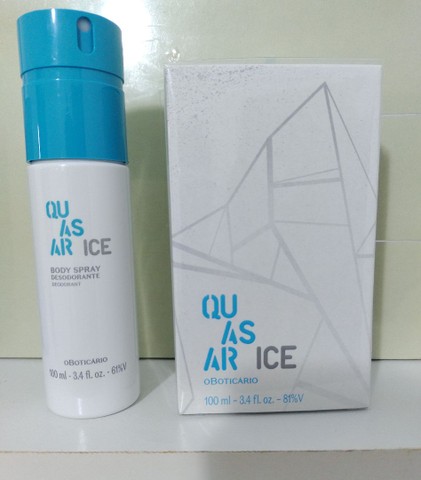This image features a promotional setup for a body spray product named "Quasar Ice." Displayed on a white or off-white shelf in front of a light gray wall, the setup includes a blue and white cylindrical bottle of body spray on the left and its corresponding box on the right. The spray bottle, with its top 40% in blue and bottom 60% in white, prominently features the product name "Q-U-A-S-A-R, ice" - "Quasar" written in blue on three lines and "ice" in gray. Below the product name, in smaller gray text, it reads "body spray, deodorant" and "Obiticario," along with the size "3.4 fluid ounces, 61% V". The vertical rectangular box, predominantly white with gray graphics, mirrors the branding on the bottle. It also states "Quasar Ice," with "Obiticario" and the volume "100 milliliters, 3.4 fluid ounces, 81% V" indicated below. The cohesive design elements such as the glacier graphics on the box and consistent color scheme emphasize the product's branding.